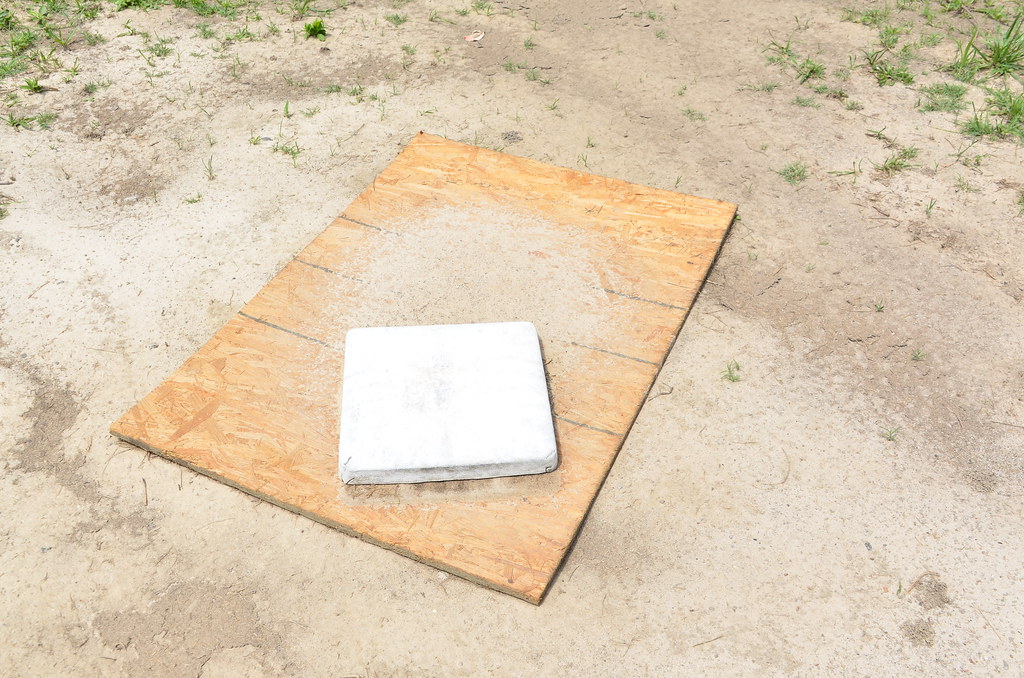The photograph, taken outdoors in an arid environment with a predominantly light brown dirt ground and sparse patches of grass, features a central wooden plank, resembling a piece of plywood, laying flat. The wood is golden-brown with three distinct grey or black vertical lines drawn on it, and it shows signs of wear suggesting it may have been sanded or used for some other abrasive activity. On top of this wooden plank sits a small, square, white cushion that appears dirty with grey stains. The scene includes minimal greenery in the upper left and right corners, likely local shrubbery or succulents, adding a touch of green to the otherwise sandy and beige landscape.